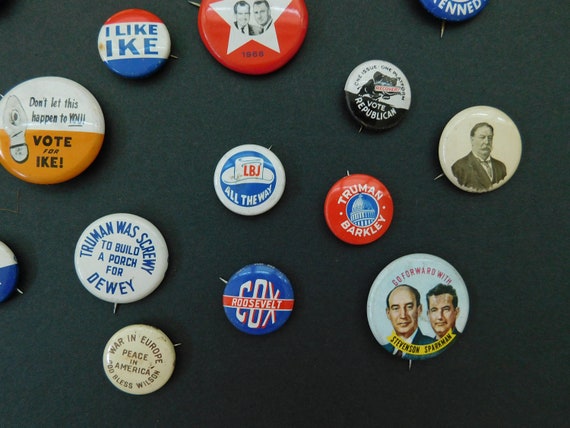This vibrant indoor close-up image showcases a collection of about a dozen vintage campaign buttons, likely spanning from the late 50s to the 60s, displayed on a dark background, possibly black or dark green felt. The buttons, which vary in size from a quarter to a half dollar, feature an array of political slogans and images from presidential campaigns. Among the prominent designs are "I Like Ike," "Truman Barkley," "Vote Republican," "LBJ All the Way," and a supportive Roosevelt button. The colors on the buttons include red, white, blue, orange, and cream, providing a vivid contrast against the backdrop. The buttons are laid out in a non-symmetrical but upright fashion, making the text and images easily readable. This photograph, likely taken from an aerial view or with a photo stand, aims to highlight the fine condition and diverse collection of these metallic campaign artifacts.